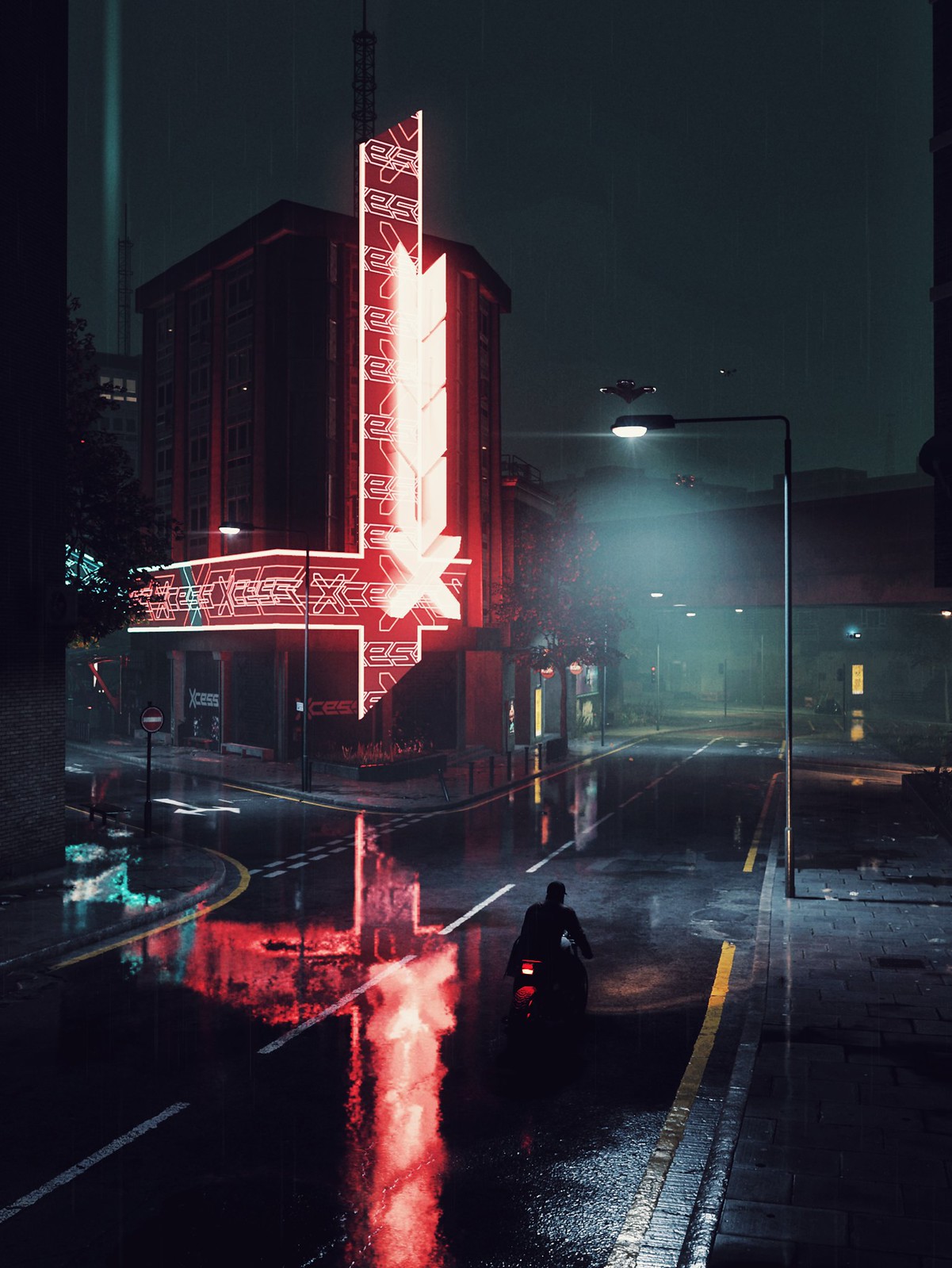This highly detailed image, likely from a modern, high-quality video game, depicts a dramatic nocturnal cityscape. The setting is shrouded in darkness, suggesting a blackout, with the only illumination coming from vivid neon signs and streetlights. Dominating the scene is a tall building that wraps around the intersection, adorned with a large, bright red neon sign that reads "XCESS," extending vertically at the corner and horizontally across the first floor.

The viewer's eye is drawn to the intricate reflections of the neon lights in the rain-slicked street, enhancing the authenticity and realism of the scene. Central to the image is a black asphalt road with distinct white and yellow lane markings, flanked by multiple lanes, one of which prominently features a solid yellow line on the right.

A man clad entirely in black, including a black baseball cap, rides a motorcycle through the wet intersection. The right edge of the image includes detailed brickwork, adding texture and depth. High above, drones or drone-like planes hover in the dark grayish-green sky, monitored by a distinct beam of light in the top left corner.

Additionally, a bridge emerges from the right and spans towards the center of the image, while a streetlamp mounted on a black pole casts a bright light on the road below, further enhancing the atmospheric tension. The image, reminiscent of the video game Watch Dogs, showcases an impressive blend of realism and artistic flair, capturing the moody ambiance of a rain-soaked, neon-lit urban environment.